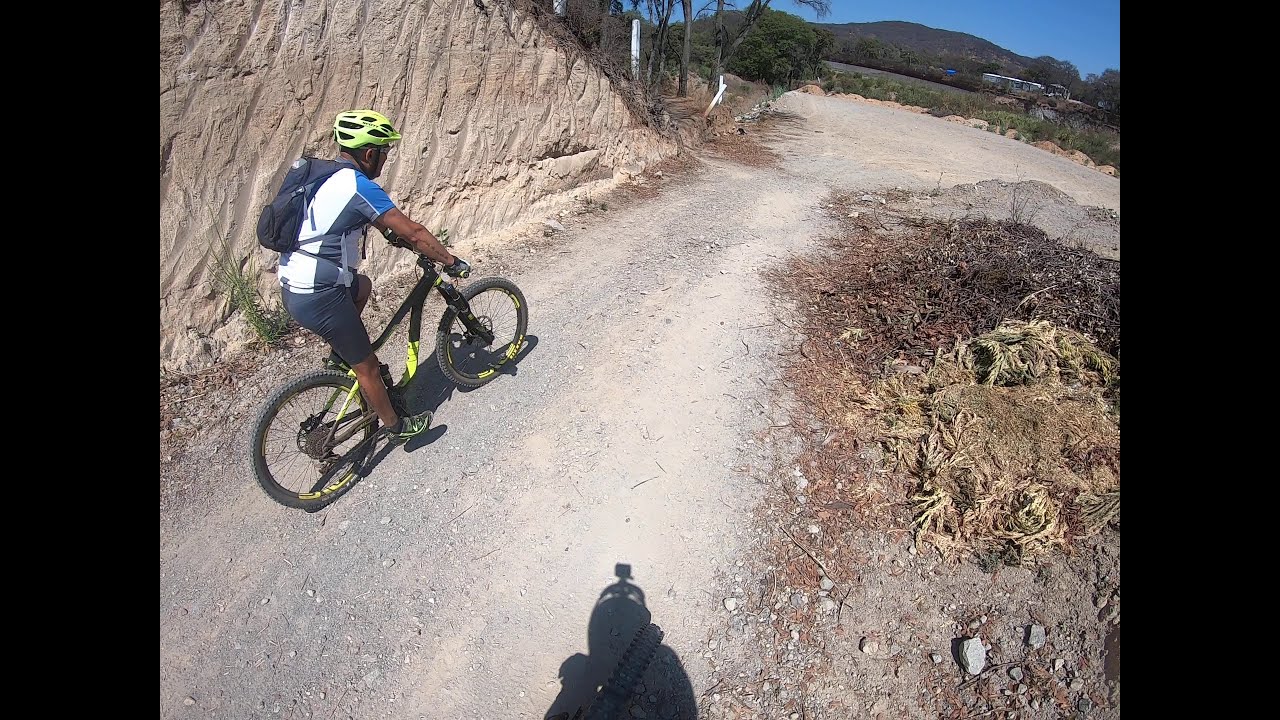In this photograph, we see a man biking on a dry, dusty dirt trail that has a few scattered stones and gravel. He is wearing a lime green helmet and a short-sleeved shirt, predominantly white with dark gray sides and a bright royal blue sleeve. The man has dark skin and a dark-colored backpack. His mountain bike is black with neon yellow accents. He faces towards the top right of the image, pedaling uphill on a slight incline. The trail is situated in a rugged, dry landscape with a pinkish beige cliff to the left and decayed plants alongside the path. In the distance, there is a lush green mountain and clear blue skies. A second rider's shadow, cast centrally in the frame, indicates that the photograph was taken with a helmet-mounted GoPro. The sun is high, and the scene seems to be bathed in daylight. Beyond the rider, the trail appears to intersect with another path, suggesting an upcoming clearing or rest area.